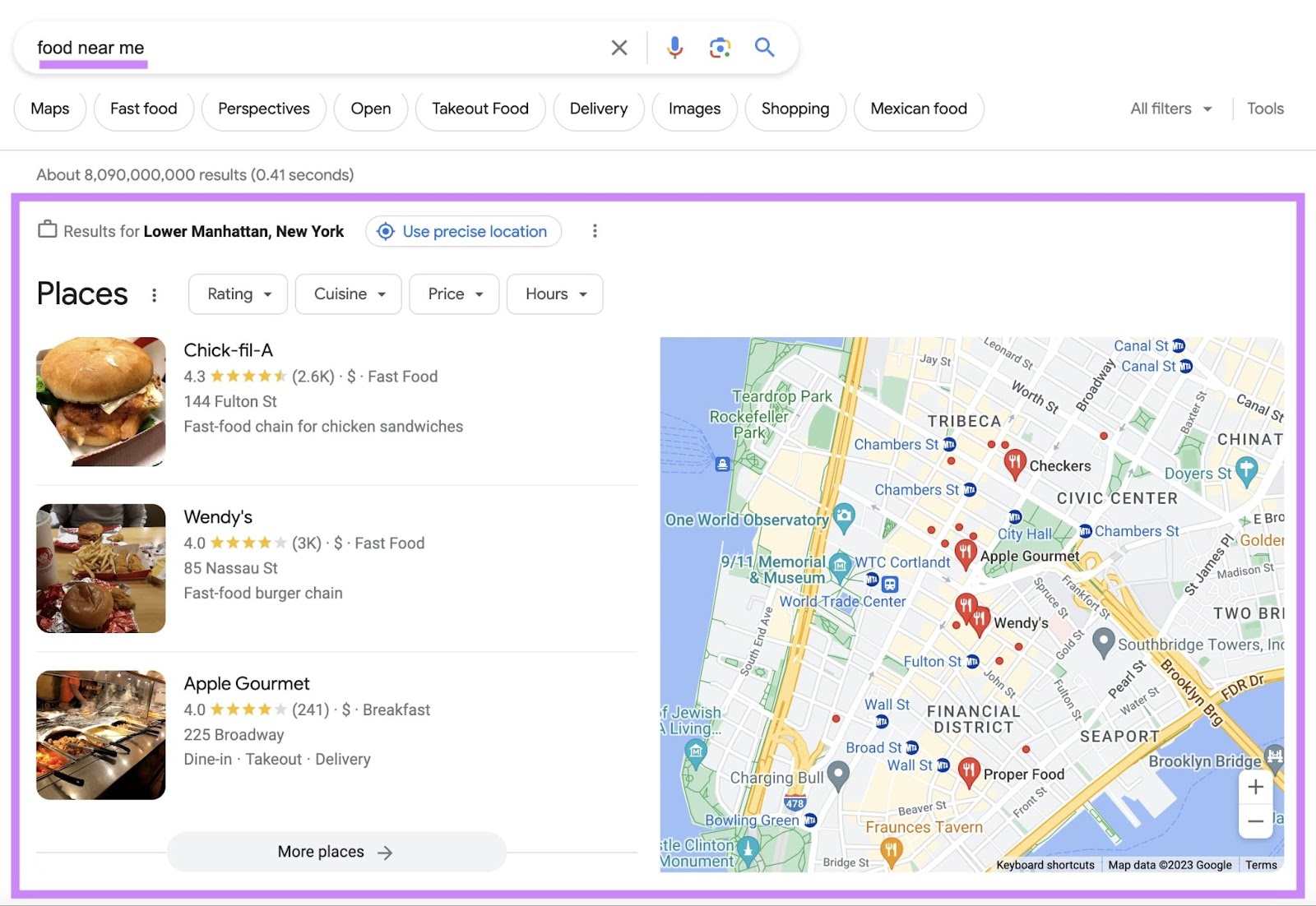The image displays a Google search results page with "food near me" typed into the search bar. At the top, several tabs are visible, including Maps, Fast Food, Perspective, Open, Take Out Food, Delivery, Images, Shopping, and Mexican Food. The search results specifically pertain to Lower Manhattan, New York. There's an option to "Use precise location" to refine the search results even further. Featured places in the list include Chick-fil-A, Wendy's, and Apple Gourmet, with Chick-fil-A notably having a rating of 4.3 stars. Additionally, there's an option to view "More places." On the right side of the screen, there's a map showing various locations, including highlighted bridges and areas surrounded by water.